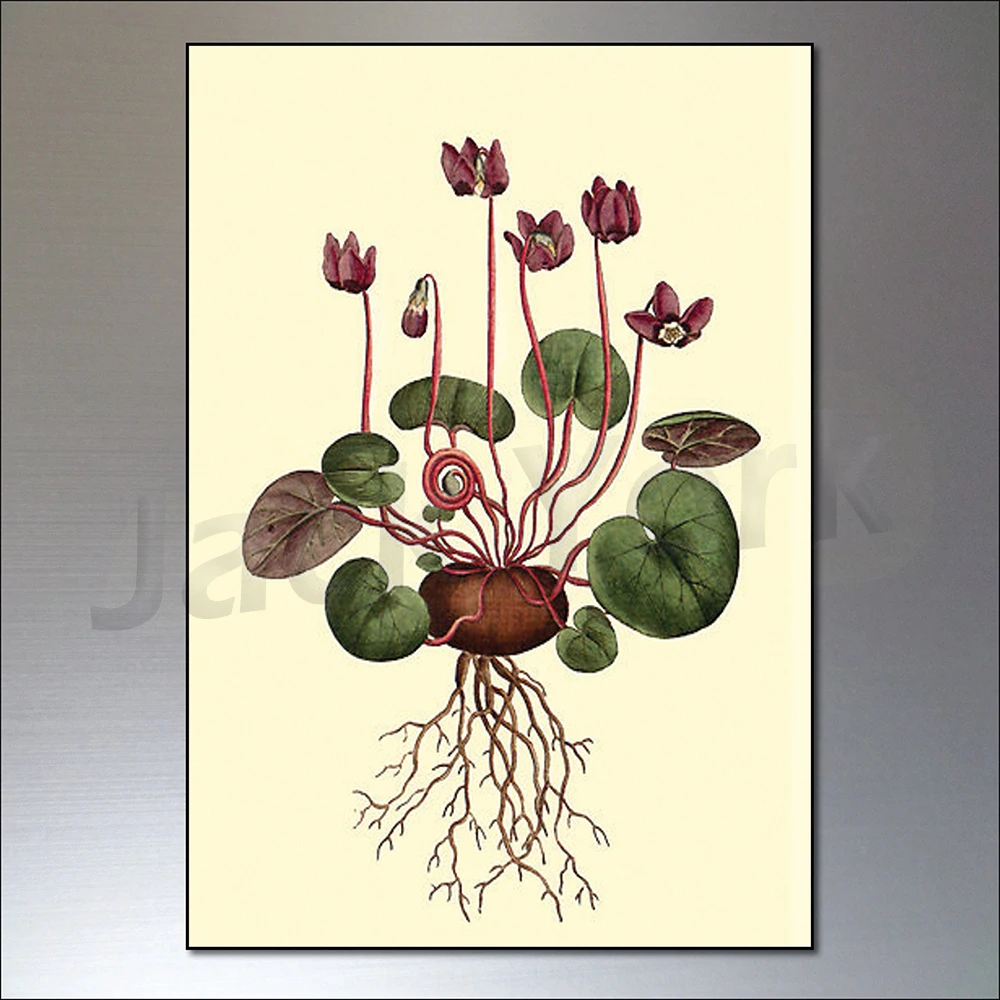The image is a detailed drawing of a unique plant set against a beige, cream-colored background, with the entire piece positioned on a gray backdrop. Across the middle of the picture, faint green letters are superimposed, including discernible letters like a capital J, A, a Y in the center, and an R at the end. The plant itself features a maroon, tomato or pincushion-shaped base with multiple maroon roots extending downward. From this base, several reddish stalks rise upward, each supporting tendrils adorned with green leaves and maroon flowers. The flowers, some of which are unopened, have distinctive white centers, and one exhibits a white, curlicue-like growth emerging from it. The illustration's composition, reminiscent of botanical art found in a museum, showcases a harmonious blend of colors and intricate natural details.